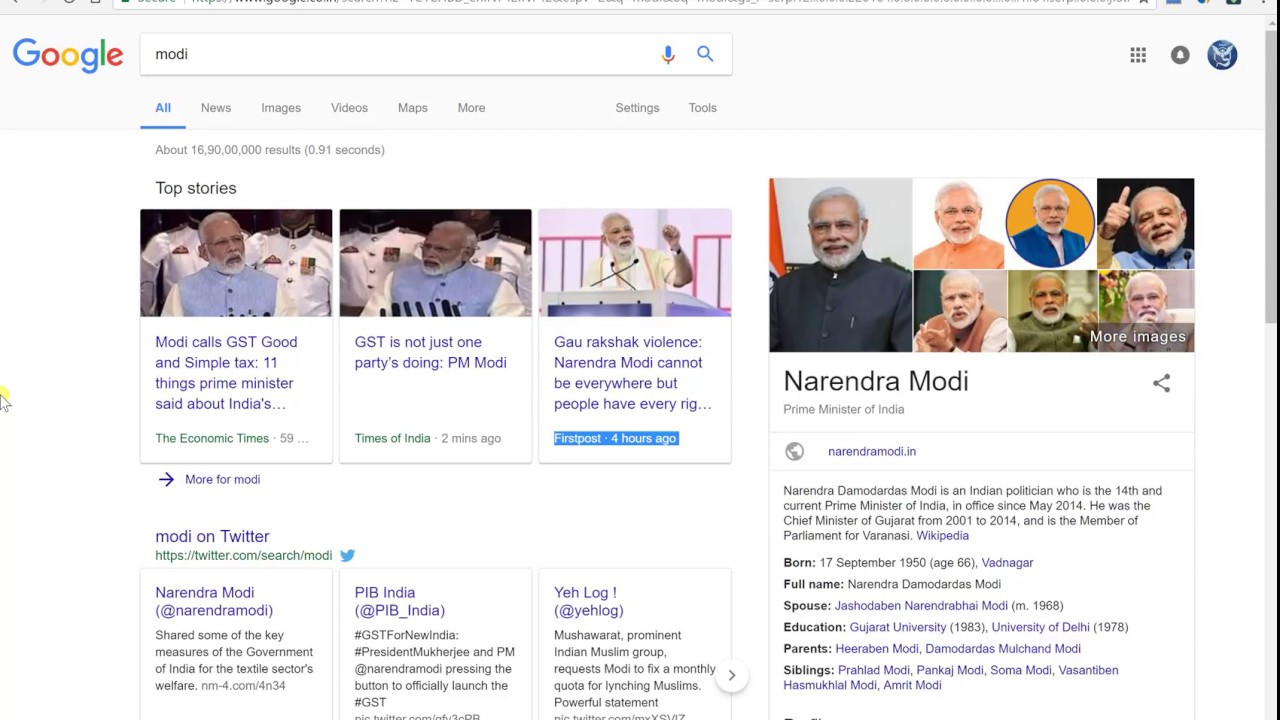This image is a screenshot of a Google search results page displayed on a computer screen. At the top left corner, the word "Google" is prominently shown next to a search bar with "MODI" typed into it. Just below the search bar, various categories are listed, including "All," "News," "Images," "Videos," and "Maps," with the "All" category highlighted. 

Beneath the categories, the heading "Top Stories" is visible, displaying three news thumbnails. All three images feature an African-American man with white hair and a white beard. The titles of the articles are:

1. "Modi Calls GST 'Good and Simple Tax': 11 Things Prime Minister Has Said About India"
2. "GST Is Not Just One Party's Doing, P.M. Modi."
3. "Gaurakshak Violence: Narita Modi Can't Be Everywhere But People Have Every Right."

On the right side of the screen, a pop-up information box provides detailed information on Narita Modi, identified as the Prime Minister of India. This box includes biographical details such as his birthdate, full name, spouse, education, parents, and siblings. Additionally, towards the bottom left corner of the screen, there is a section labeled "Modi on Twitter," which includes his Twitter handle.